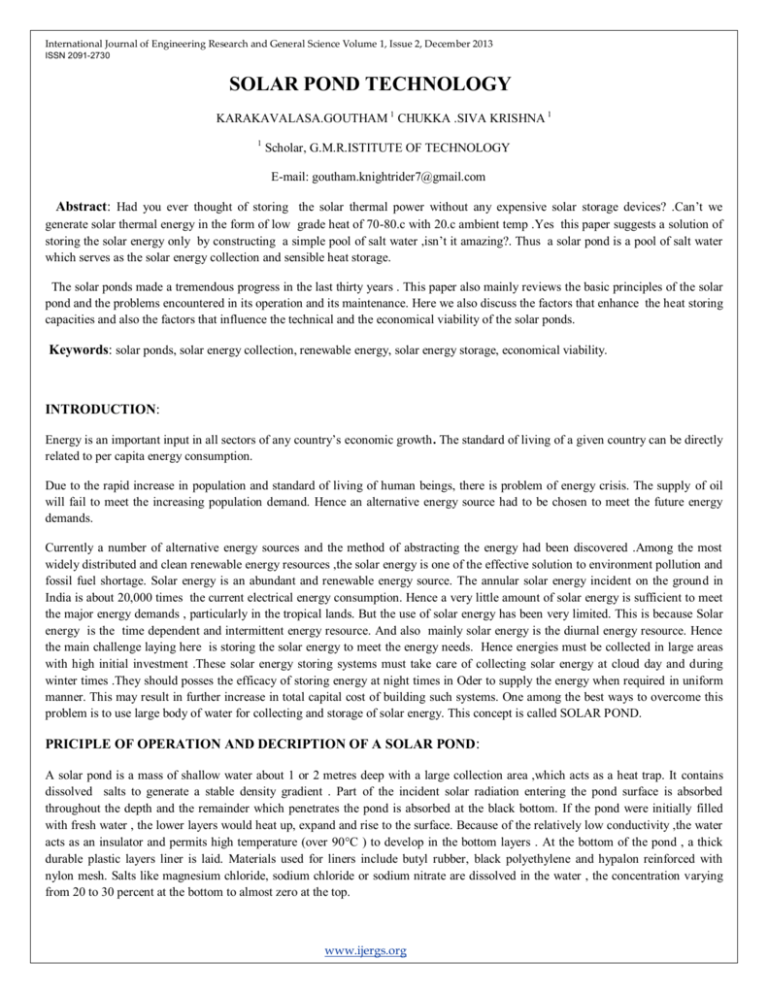This document features a detailed layout on a white background with black or gray text, all encompassed by a light gray rectangular border. At the bottom, highlighted in bright blue and underlined, is the website link: [www.jergs.org](http://www.jergs.org).

In the upper left-hand corner, in very tiny gray text, the header reads: "International Journal of Engineering Research and General Science, Volume 1, Issue 2, December 2013," followed by an ISSN number: "2091-2730."

Centered on the page in large, bold black text is the title: "Solar Pond Technology." Below the title, the authors' names and an email address are listed.

The section begins with the word "Abstract" in bold black text, followed by two gray paragraphs detailing the abstract. Subsequent to the abstract is the "Keywords" section in bold black text, listing the terms: "Solar Ponds, Solar Energy Collection, Renewable Energy, Solar Energy Storage, Economical Viability," all in gray text.

The next section is titled "Introduction" in bold, capitalized black letters and consists of three paragraphs. Following this, another section titled "Principle of Operation and Description of a Solar Pond" appears in bold, capitalized black letters, although there might be a typographical error in the title.